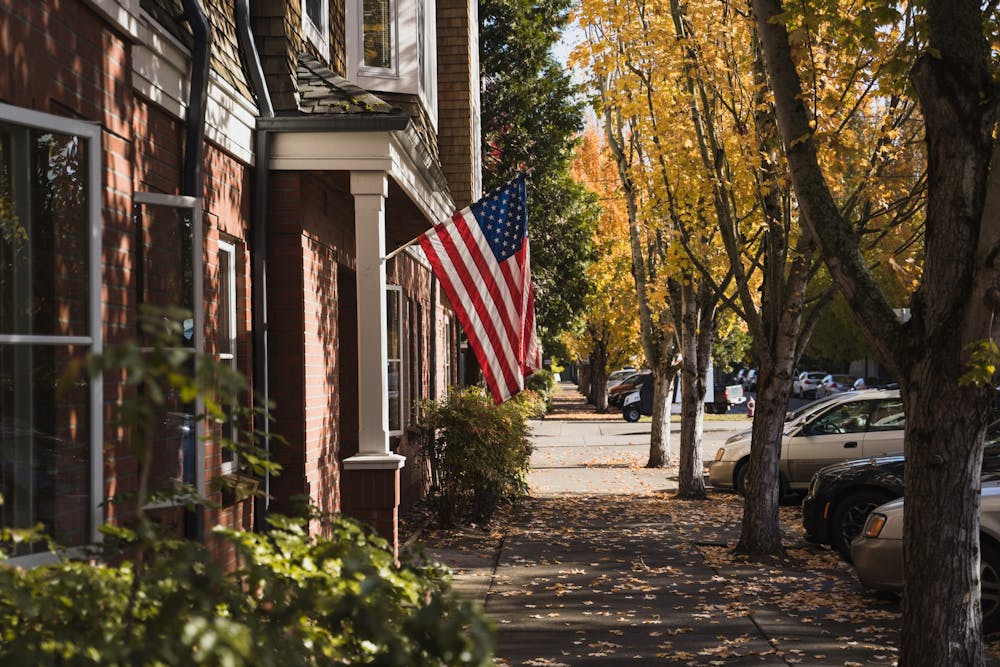The color photograph captures a sunny fall day on a sidewalk adorned with both green and autumnal yellow leaves. To the right of the sidewalk, there is a row of trees displaying a mix of green, yellow, and red foliage, and the shadows cast by these trees darken portions of the walkway, which is also scattered with fallen leaves. On the left stands a red brick building with white pillars, identified as a home or possibly an apartment or storefront. An American flag is prominently displayed, billowing in the wind. Further to the right, beyond the row of trees, several cars are parked along the street. The overall lighting suggests it is a bright day with crisp shadows and vibrant colors.